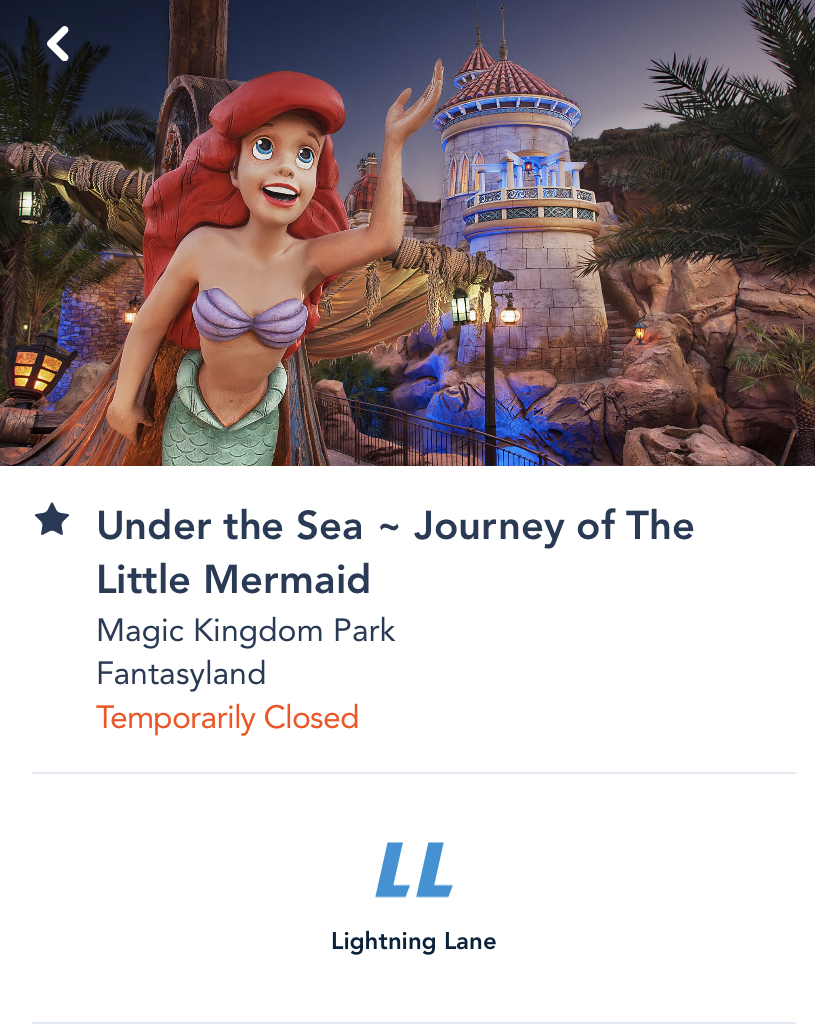This image is a screenshot from an unspecified web page, featuring a color photograph of a Disneyland attraction. The focal point of the photograph is a detailed statue of Ariel from "The Little Mermaid." Ariel is depicted with flowing red hair and expressive blue eyes. She looks upwards with a joyous smile, her left hand raised high in an animated gesture. She is dressed in her iconic purple seashell bra, and her green mermaid tail, partially cut off by the bottom edge of the photograph, is visible.

In the background, the mast of a ship adds a touch of maritime adventure, while to Ariel's right, a lighthouse stands surrounded by a cluster of rocks, contributing to the seascape theme of the attraction. Below the photograph, text indicates the name and status of the attraction: "Under the Sea, Journey of the Little Mermaid, Magic Kingdom Park, Fantasyland, Temporarily Closed," with "Temporarily Closed" highlighted in orange letters. At the bottom of the screenshot, two bold blue letters, "LL," stand for Lightning Lane, accompanied by smaller black text.

Notably, the image includes no real people, animals, birds, fish, or automobiles, maintaining an entirely animated and whimsical atmosphere.